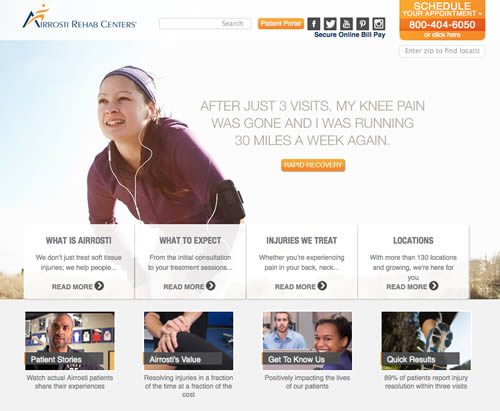An image from the Airsoft Rehab Centers website features a detailed and inviting interface designed to engage visitors. 

At the top, the Airsoft Rehab Centers logo is prominently displayed in blue capital letters with a touch of orange decoration. Adjacent to the logo on the right, there's a search bar, followed by an orange-background button labeled "Patient Portal." Social media icons for Facebook, Twitter, Pinterest, and Instagram are aligned next to this, and below them is a link for "Secure Online Bill Pay." An orange box to the far right reads "Schedule Your Appointment" alongside the contact number 800-404-6050 with a prompt to "Click Here." Beneath this is the instruction to "Enter VIP to Find Location."

Dominating the main part of the image is a large white box with a hint of light blue on the left, possibly representing the sky. In this area, a middle-aged Caucasian woman smiles warmly, adorned with a headband and earbuds. She wears a maroon athletic jacket reminiscent of a tracksuit, suggesting she has been running. The accompanying text states in bold capital letters, "After just three visits, my knee pain was gone. I was running 30 miles a week again." Beneath this, in smaller text, it reads "Hard recovery."

Below the main image are four informative boxes, each featuring a Read More link:
1. "What is ARISTI?" - "We don't just treat soft tissue injuries, we help people."
2. "What to Expect" - "From Initial Consultation to your Treatment Sessions."
3. "Injuries Retreat" - "Whether you're experiencing pain in your back, neck, etc."
4. "Locations" - "With more than 130 locations and growing, we're here for you."

At the bottom, there are thumbnails for four videos providing deeper insights:
1. "Patient Stories" - Featuring a gentleman in the thumbnail.
2. "ARISTI's Value" - Showing someone’s hands and forearms, possibly a woman.
3. "Get to Know Us" - Depicting a young Caucasian man in a blue shirt and an African-American young lady also in a blue shirt.
4. "Quick Results" - The thumbnail shows a tree and the back of someone's sneaker, suggestive of someone mid-run.